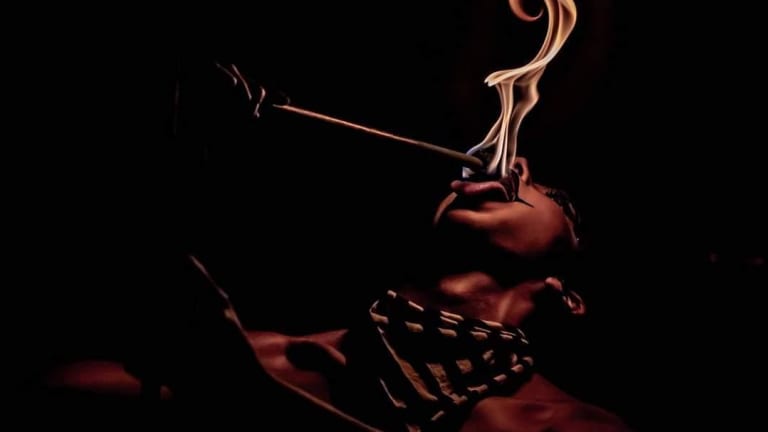The image captures a dramatic scene of a fire-breather performing against a pitch-black background, reminiscent of a nighttime setting. The only source of illumination is the vivid, golden flames emanating from a sponge at the end of a stick, which the performer appears to be swallowing. The performer, who has darker brown skin, has their head thrown back, mouth open wide, and tongue outstretched, creating an intense and captivating visual. They are adorned with a white and black striped scarf or bandana around their neck, adding a striking contrast to the dim surroundings. The performer, possibly a woman indicated by thick eyelashes, does not appear to be wearing a shirt, and their hands are barely visible due to the shadowy lighting. The mesmerizing flames cast dynamic shadows, highlighting the performer's facial features and the outline of their head, neck, and shoulders, emphasizing the bravery and skill involved in the act of fire-breathing.